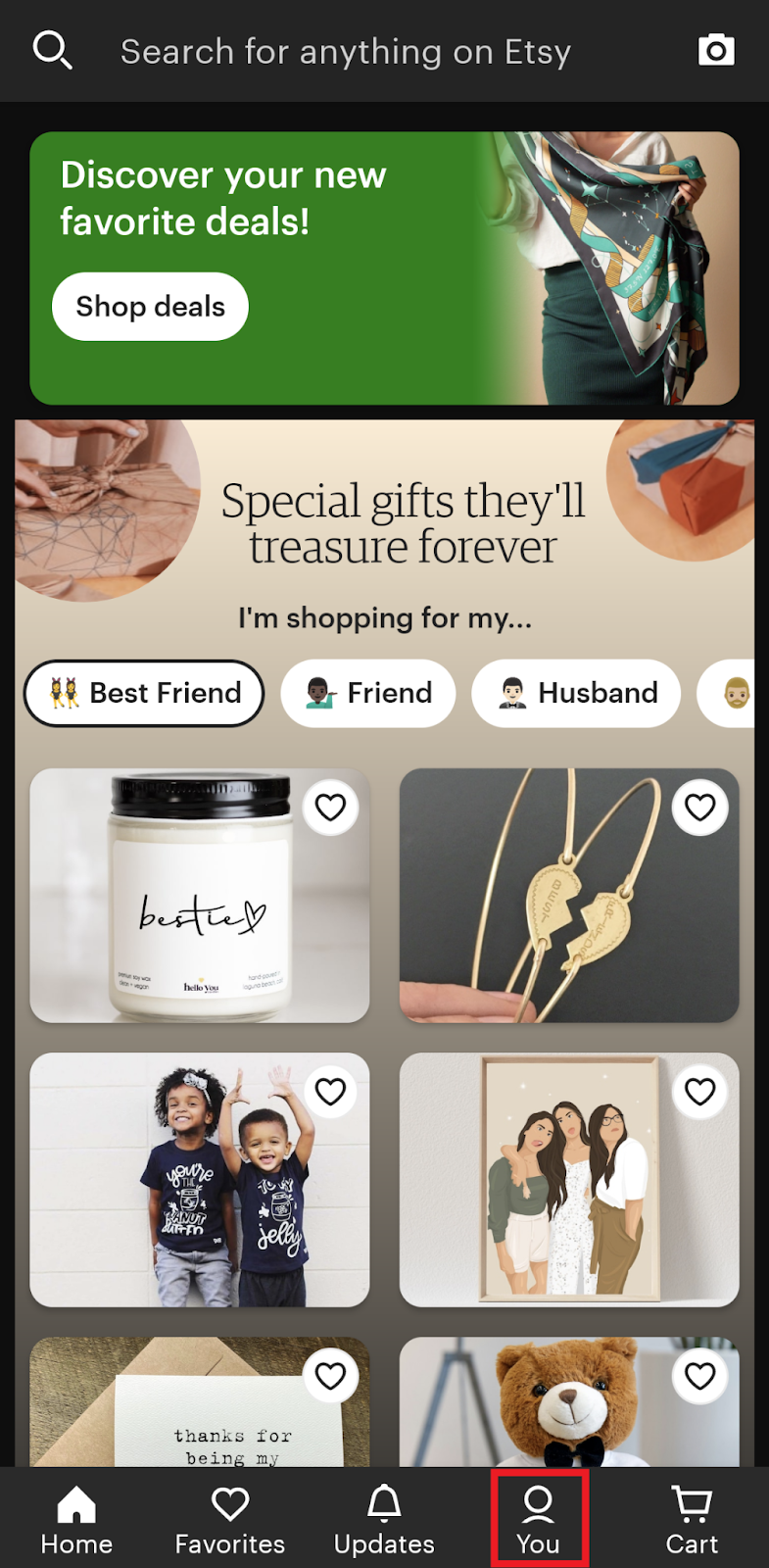This screenshot displays a mobile application with a sleek and modern user interface. The background is predominantly black, creating a striking contrast with the dark gray header at the top. On the left side of the header, a white magnifying glass icon is prominently featured, followed by white text that reads, "Search for anything on Etsy." There is some negative space, then a white camera icon appears to the right.

Beneath the header, the black background continues, displaying two distinct tiles. The first tile occupies most of the frame's width and has rounded corners. It features a gradient transition from a solid green color on the left to a photograph on the right. The photograph showcases a person in a white shirt and green skirt. In the top left corner of this tile, bold white text reads, "Discover your new favorite deals!" Below this, a white, pill-shaped button with black text inside reads, "Shop deals."

The second tile, separated by a thin black line, is almost full-frame in both width and height. It boasts a beige to dark gray gradient background, with beige at the top and dark gray at the bottom. At the top center, black text announces, "Special gifts they'll treasure forever." Beneath this, smaller bolded text reads, "I'm shopping for my..." with an ellipsis. To the left, a round photograph shows a person tying a brown paper package with a bow, and to the right, another photograph displays a wrapped brown paper package. Below the text, several white, pill-shaped buttons with rounded corners are present. The first button has a black outline and contains black text that reads, "Best friend."